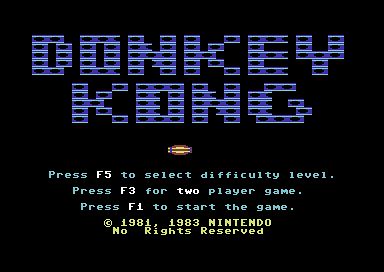The image depicts an old video game start screen with a black background. At the top, "Donkey Kong" is displayed in pixelated blue and black letters, making it somewhat difficult to read. Below, there are two lines of orange lights in the center. Underneath those lines, green text instructions are presented: "press F5 to select difficulty level," "press F3 to play your game," and "press F1 to start the game," with the F keys highlighted in white. Some of the text appears in green, while the copyright notice at the bottom— "1981, 1983 Nintendo, no rights reserved"—is in yellow. The overall text appears blurry with lines going through it, giving a vintage look, characteristic of early video game graphics.